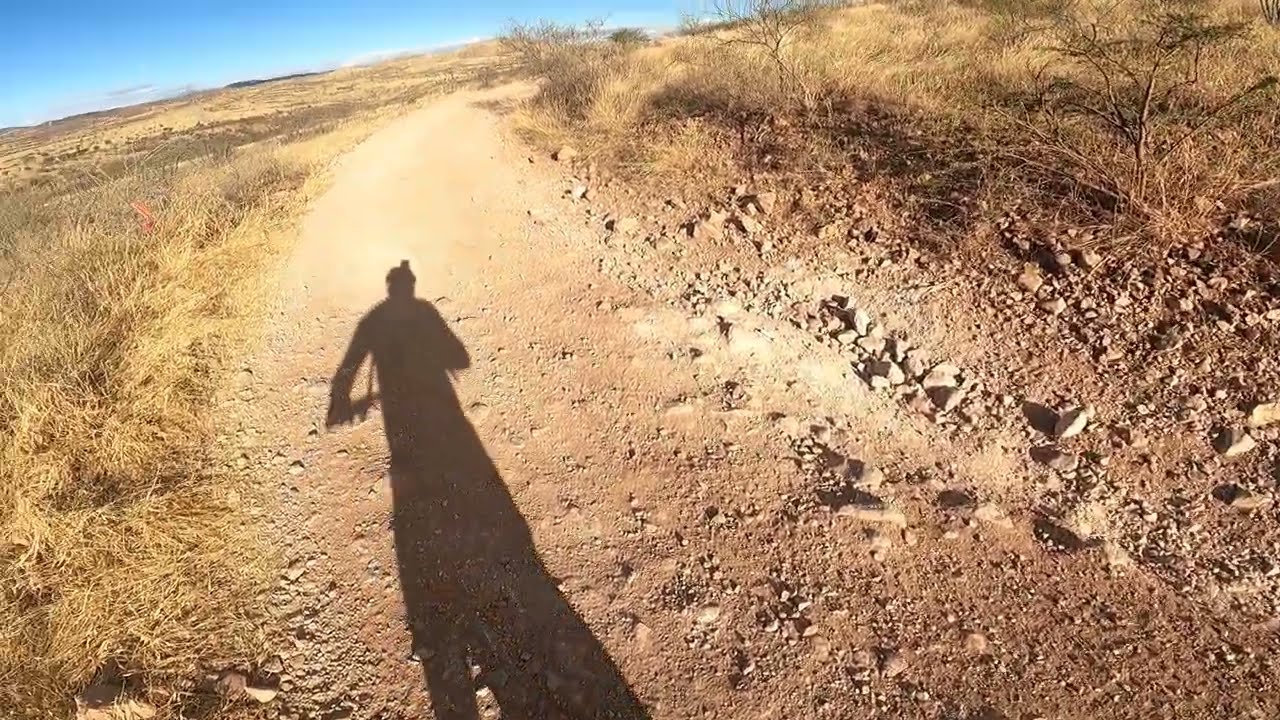The image is a daytime outdoor photograph featuring a rugged, desert landscape with a dirt path carving through it. The sky in the upper left corner transitions from a brilliant blue to lighter hues near the horizon. Pale yellow and golden dried-out foliage dominates both the upper right and lower left areas. Along the rocky path, which stretches from the lower right towards the center and then curves upward to the left, the shadow of a cyclist is cast. The cyclist is wearing a helmet with a mounted camera, which is evident from the elongated shadow indicating the sun is low, either early in the morning or late in the afternoon. The handlebars and part of the thin wheel of the bike are visible, enhancing the sense of movement along the dusty trail.